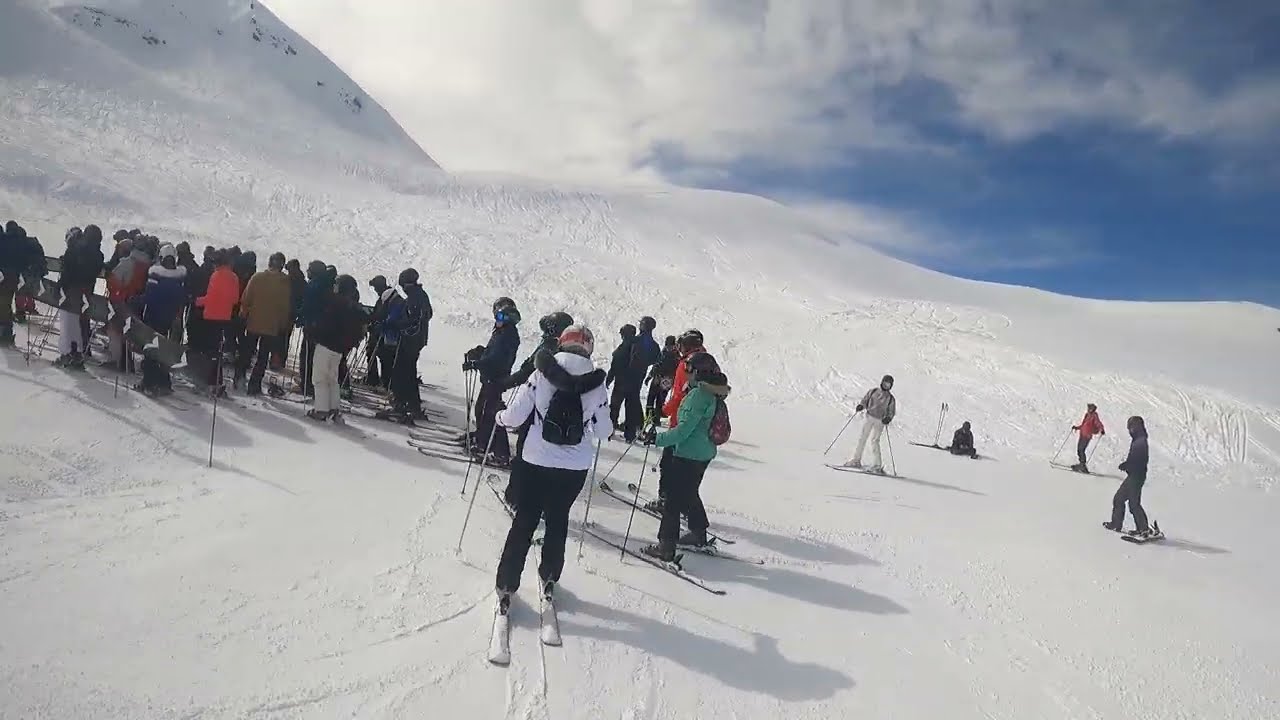This photograph captures a bustling ski slope blanketed in pristine white snow under a vibrant blue sky dotted with cumulus and cirrus clouds. The scene centers on a slight incline, where numerous skiers are gathered, predominantly towards the left side of the image. These skiers are attired in colorful winter clothing, including jackets in shades of white, green, red, blue, and black, as well as winter hats and possibly ski masks. Their skis, which often drag or bear patches of snow, carve numerous tracks into the snow-covered ground. In the very center, a woman in a white coat with a black fur-lined hood and black pants stands beside two skiers dressed in green and black and red coats, respectively. Around them, at least 30 to 40 skiers are either queued up, waiting for their turn to descend, or moving slightly in line for the ski lift, creating a lively, anticipatory atmosphere. In the distance, hills of varying steepness frame the scene on both sides, enhancing the depth and inviting the viewer into this wintry landscape.